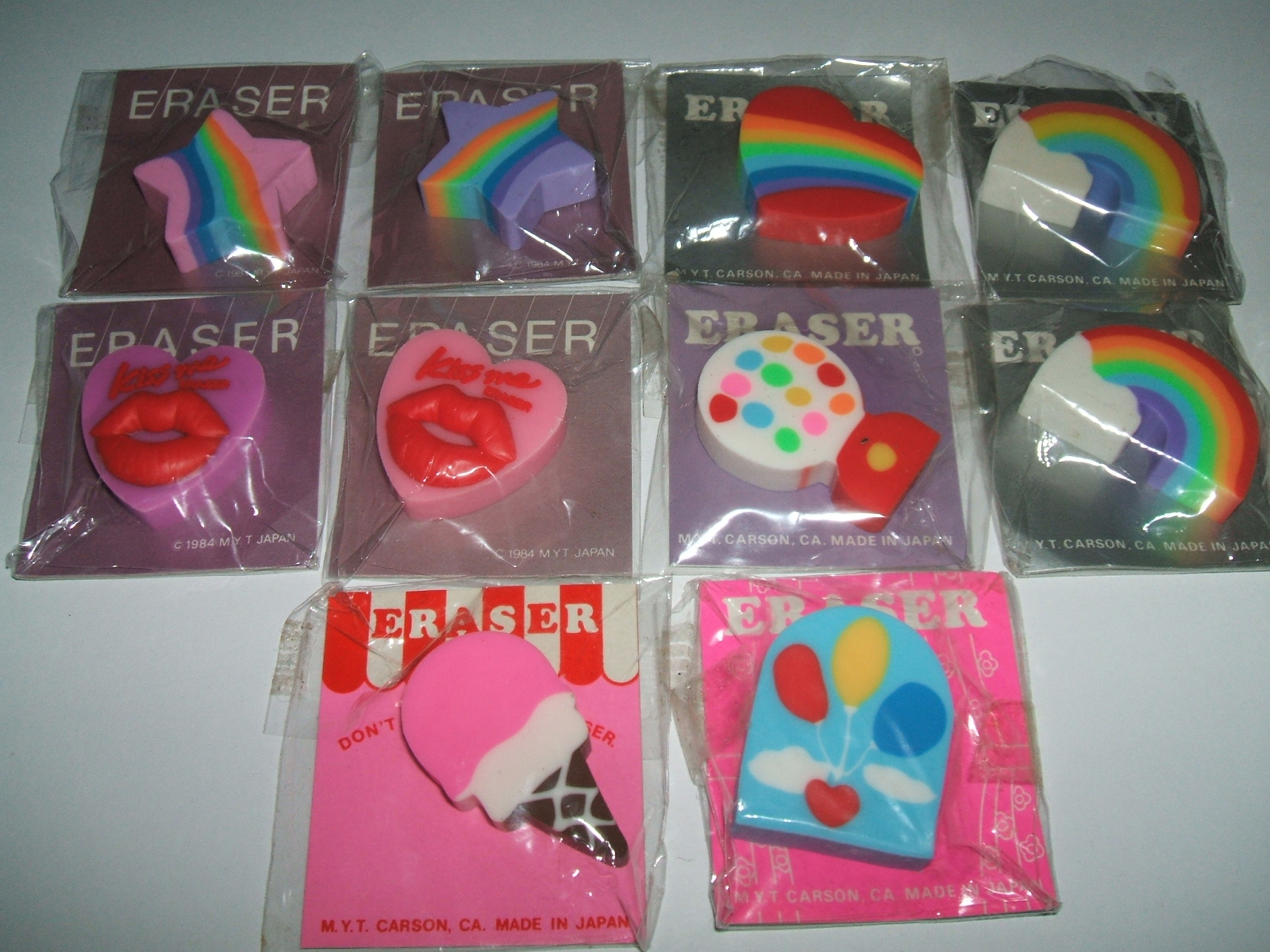This indoor color photograph provides a close-up view of ten brightly colored, fun-shaped erasers individually wrapped in square plastic packages. The erasers are laid out on a white surface, possibly a table or shelf, and are arranged in three rows: the first two rows each contain four packages, and the bottom row contains two. Each eraser package prominently displays "ERASER" at the top, with "MYT Carson California" and "Made in Japan" at the bottom.

The detailed arrangement from top to bottom is as follows: 

- **Top Row:** A blue star with a rainbow, another star with a rainbow, a heart with a rainbow design, and a rainbow.
- **Middle Row:** Two hearts with red lips on them, a gumball machine, and another rainbow.
- **Bottom Row:** An ice cream cone with pink ice cream and a balloon-shaped eraser.

Overall, the variety of shapes includes stars, hearts, rainbows, a gumball machine, an ice cream cone, and a balloon, emphasizing the erasers' playful and colorful designs.